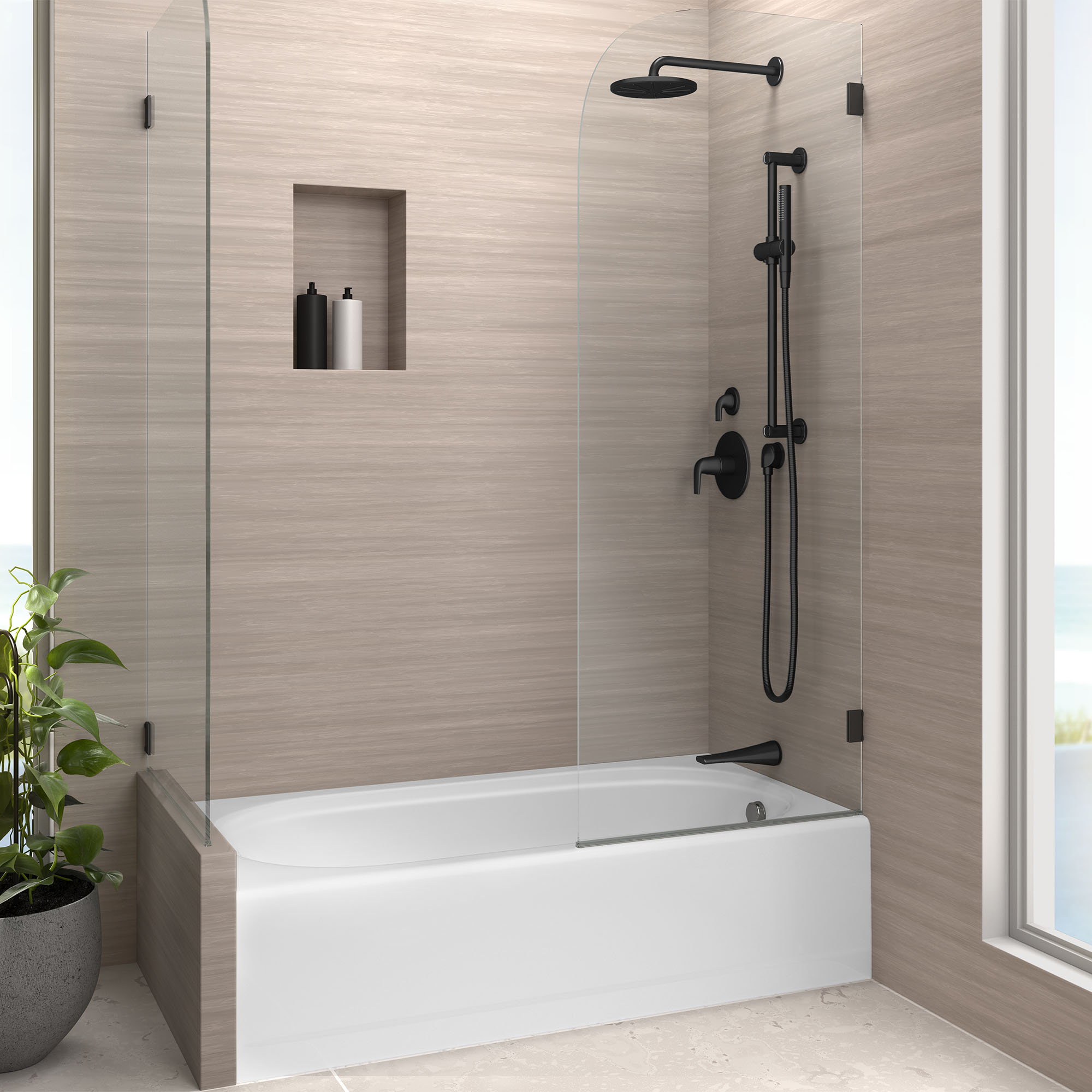The image depicts a modern bathroom with a porcelain white bathtub-shower combination, designed with clean, angular lines and built into the floor. The surrounding walls are beige with horizontal lighter and darker streaks, likely resembling wood grain. At the front of the bathtub is a silver knob, and above it, a black faucet and a shower hose looping downward from the wall connect to a vertically aligned black metal rod. The shower features a large black shower head at the top and two black handlebars, one smaller than the other, positioned to the left. A recessed rectangular shelf in the shower wall holds black and white bottles of shampoo or hair products. The shower enclosure consists of two clear glass panels, one on the left and one on the right, held in place with black metal fittings, leaving an open entryway. To the right of the tub, there's a floor-to-ceiling window, partially visible, suggesting a high-ceiling room. At the foot of the tub sits a large leafy green potted plant in a gray pottery planter, and the floor is a tan or beige color.